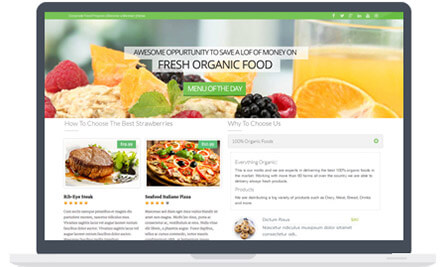The webpage of an unidentified company features a vibrant header image displaying a plate of assorted fresh fruits including raspberries, pineapple, and blackberries, accompanied by a picture of a glass of orange juice to the right. Prominently, the webpage advertises an "awesome opportunity to save a lot of money on fresh organic food". Key sections of the site include links titled "Menu of the Day", "How to Choose the Best Strawberries", and "Why Choose Us". Below, the content becomes blurry, but several elements are discernible: an image of a ribeye steak labeled with five-star ratings, a partially legible description beneath a picture of a pizza rated four out of five stars, and a dropdown menu labeled "100% Organic Foods". The remaining text is too small and indistinct to be read clearly. The image contains no people, animals, birds, fish, insects, buildings, automobiles, bicycles, or airplanes.